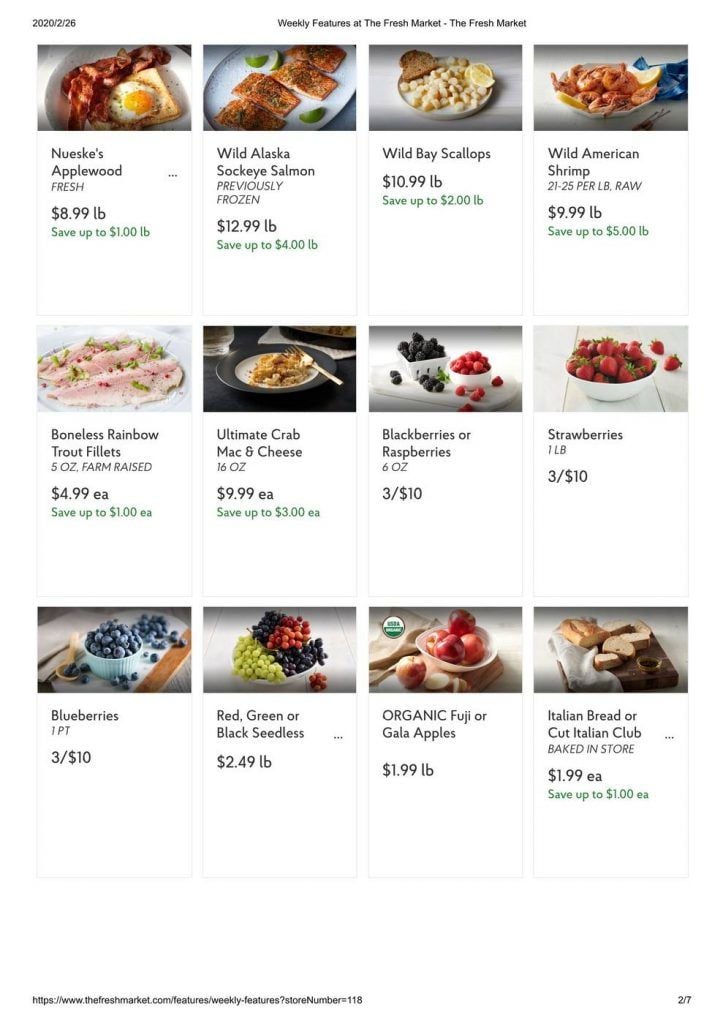This image depicts a webpage showcasing the food products offered by a market. In the upper left-hand corner, faint but visible, is a date that appears to read either "2020-26" or something similar.

Prominently displayed in the center of the page is a banner with the text, "Weekly Features at the Fresh Market - The Fresh Market." Beneath this heading are three rows of images, each featuring four products, along with their respective prices and saving information.

- **NuZex Applewood Fresh**: Priced at $8.99 per pound with a savings offer of up to $1 per pound, highlighted in green. The accompanying image appears to show a breakfast platter with bacon and eggs on toast.
- **Wild Alaska Sockeye Salmon**: Previously frozen and available at $12.99 per pound with savings of up to $4 per pound.
- **Wild Bay Scallops**: Listed at $10.99 per pound, offering savings of up to $2 per pound.
- **Wild American Shrimp**: Priced at $9.99 per pound.
- **Boneless Rainbow Trout Fillets**: Available for $4.99 each.
- **Ultimate Crab Mac and Cheese**: Priced at $9.99.
- **Fresh Berries**: Offer includes blackberries, raspberries, strawberries, and blueberries, sold in a mix-or-match format.
- **Seedless Grapes**: These include red, green, or black varieties.
- **Organic Fuji or Gala Apples**: Featured among the fresh picks.
- **Italian Bread / Cut Italian Bread**: Baked in-store, priced with a savings of up to $1 each.

The products follow a consistent layout format with pricing and saving offers clearly indicated next to each item image.